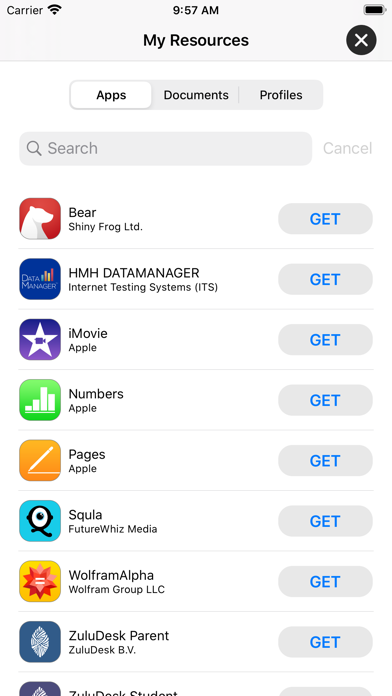This is a detailed screenshot of a mobile app interface displaying personal resources. At the top of the screen, the current time is shown as 9:57 AM. Directly below the time, there is a section labeled "My Resources," with an "X" button positioned at the top right corner on a black background. Below this section, there are three tabs: Apps, Documents, and Profiles. The "Apps" tab is highlighted in white, indicating it is currently selected.

Under the tabs, there is a search bar with the placeholder text "Search" and a "Cancel" button to the right of it. Below the search bar, a list of app icons is displayed. The first row features the "Bear" app by ShinyFrog LTD, with an icon depicting a white silhouette of a bear on a red background. To the right of this icon is a "GET" button. The second row shows the "HMH Data Manager" app, also accompanied by a "GET" button to its right.

In the third row, there is the "iMovie" app from Apple. Its icon has a purplish background featuring a white star, with a purple camera inside the star. A "GET" button is placed to the right of this icon. The fourth and final row displays the "ZuluDesk Parent" app, which also has a "GET" button to its right.